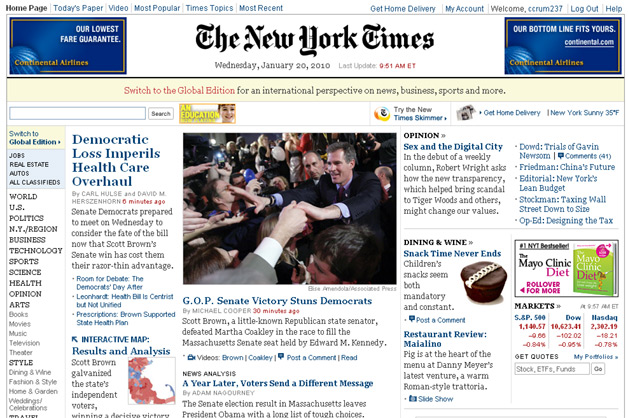Screenshot of The New York Times Home Page - January 20, 2010

This image is a screenshot of the New York Times homepage from Wednesday, January 20, 2010. The top headline prominently announces, “Democratic Loss Imperils Healthcare Overhaul,” highlighting that Senate Democrats are set to convene on Wednesday to discuss the future of the healthcare bill after Scott Brown's Senate victory, which cost them their fragile majority. The subheading elaborates, noting that Scott Brown, previously a relatively unknown Republican state senator, defeated Democrat Martha Coakley in the race to fill the Massachusetts Senate seat formerly held by Edward M. Kennedy.

Another significant headline reads, “GOP Senate Victory Stuns Democrats,” alluding to the shock and political ramifications arising from Brown's unexpected win. A feature column titled “Sex and the Digital City” is introduced, where Robert Wright explores how increasing transparency in the digital age has exposed scandals involving public figures like Tiger Woods and speculates on its potential to reshape societal values.

Additionally, a lifestyle piece entitled “Snack Time Never Ends” comments on the ubiquitous and seemingly obligatory nature of children's snacks. This snapshot captures the pressing news and cultural discussions of that day, providing a window into the concerns and interests of early 2010.